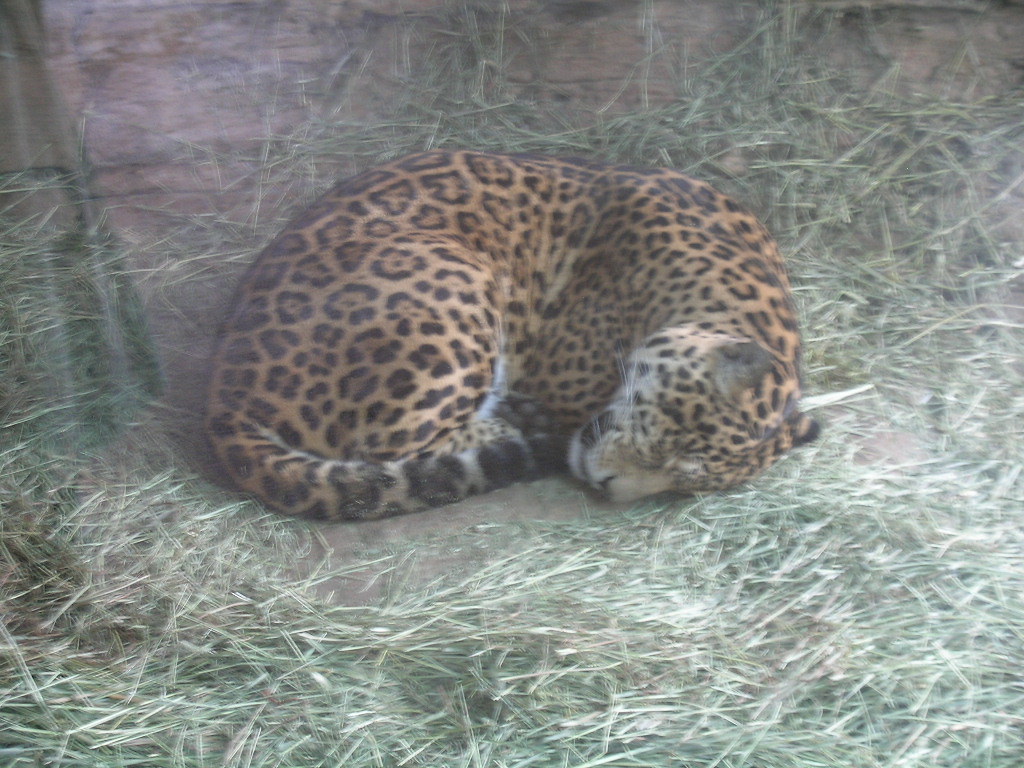In this slightly out-of-focus photograph taken inside a zoo, a majestic orange leopard adorned with an intricate pattern of black spots is seen curled up tightly in a small dirt nest. The sleepy feline is nestled against a large rock wall, surrounded by dry grass and sparse brush, giving the scene a naturalistic feel. The intimate setting captures the tranquility and beauty of the leopard in its quiet repose.